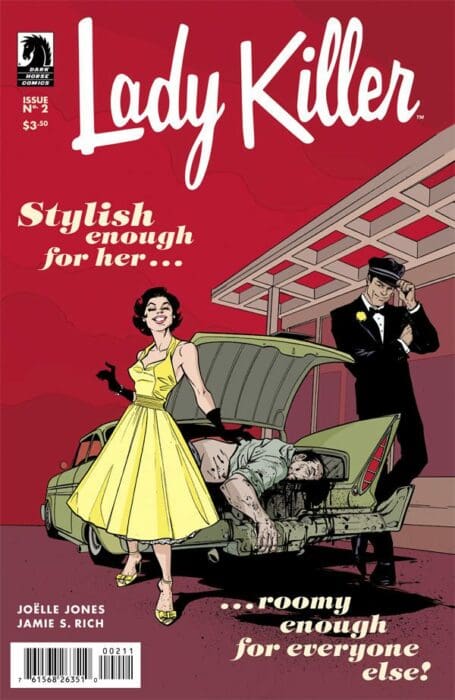The cover of Issue Number 2 of the comic by Dark Horse Comics is a vibrant and detailed illustration in a vintage style. The Dark Horse Comics logo, a black horse on a white background, is positioned in the upper left corner, alongside the issue number and price, $3.50. The title "Lady Killer" is displayed to the right in partially cursive white text. Just below, it reads "Stylish Enough for Her..."

The central image showcases a confident woman with short dark hair, dressed in a 1950s-1960s era yellow dress that flares out at the bottom, and cinched at the waist. She accessorizes with black elbow-length gloves and a bracelet on her right hand. Smiling, she stands beside a vintage green car with an open trunk. In the trunk, a man's body is partially visible, with black stains indicating blood seeping from the trunk. 

A chauffeur, also smiling and dressed in a sharp suit with a yellow flower or corsage, stands to the right of the car, tipping his cap. The backdrop features a building with pillar-supported square structures, adding to the vintage ambience. At the bottom of the cover, the copy reads "...Roomy Enough for Everyone Else." The authors, Joelle Jones and Jamie S. Rich, are credited in the lower left corner above a barcode.